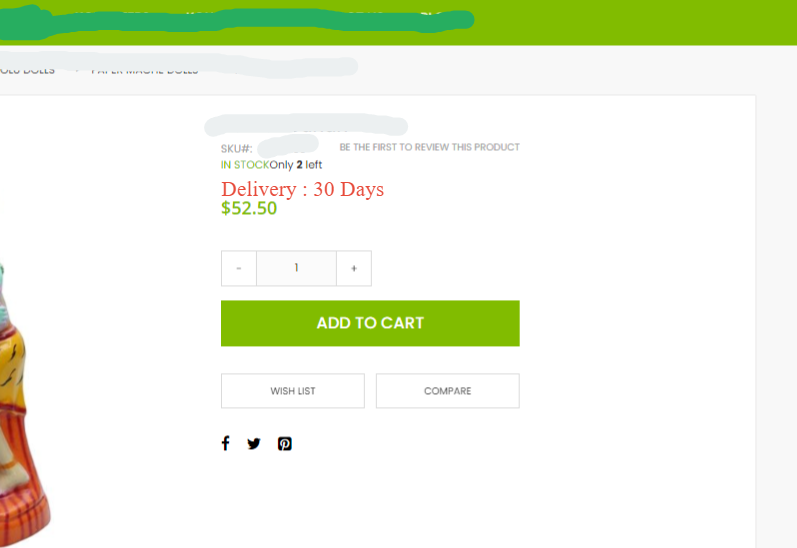The image showcases a webpage with a green header at the top, accented with blue and gray areas. Various elements are covered, contributing to a cluttered appearance. Prominent text on the page includes "SKU" followed by a pound sign, and "Be the first to review this product." The product is noted to be "In stock" with only "two left." Delivery information states "call in 30 days." The price is highlighted in red as $52.50, with quantity controls nearby: a minus sign, the number one, and a plus sign. A green rectangle button labeled "Add to Cart" is visible, accompanied by options for "Wish List" and "Compare." Social media icons for Facebook, Twitter, and Pinterest are also present. On the left-hand side, there is a partially obscured image of a ceramic figure, which appears to be wearing a yellow coat and an orange dress.